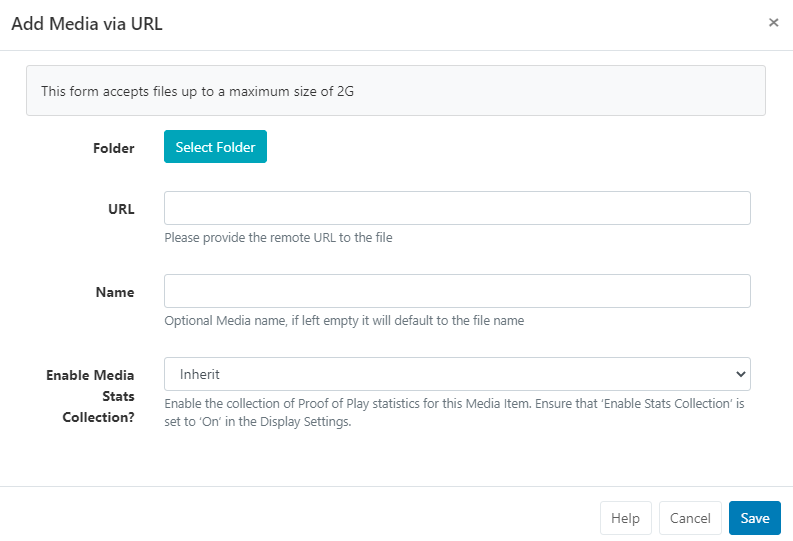The image is a detailed screenshot of a webpage form intended for adding media via a URL. The entire page features a white background with all text and form elements clearly laid out against it.

At the very top, there's a prominent instruction in black text: "Add Media via URL". Directly below this title sits a horizontal light gray line, which helps separate the heading from the form below. At the far right end of this line is a small black "X", presumably for closing the form.

Beneath the line, a light gray rectangular box contains a message in black text: "This form accepts files up to a maximum size of 2G." The capitalized "G" stands out for its emphasis on the size limit.

Following this, there is a label "Folder" in black text, next to which is a blue rectangular button with the white text: "Select Folder". Below this section, another label "URL" is presented in black text, followed by a long, empty white rectangle with a gray outline, meant for inputting the URL. Directly underneath this input box, an information line reads: "Please provide the remote URL to the file."

Further down, the label "Name" appears in black text followed by another blank input space. Under this space, an explanatory note states: "Optional media name. If left empty, it will default to the file name."

The next feature on the form is a question: "Enable media stats collection?" beside which is a drop-down menu displaying the word "Inherit". This drop-down can be customized by clicking the small arrow on its right. An additional note underneath reads: "Enable collection of proof of play statistics for this media item. Ensure that enable stats collection is set to on in the display settings."

At the very bottom of the form, three buttons are presented from left to right: "Help", "Cancel", and "Save". The "Help" and "Cancel" buttons are white with black text, indicating they have not been clicked. The "Save" button, in contrast, is blue with white text, indicating it has been clicked or selected.

This meticulously detailed form is designed to assist users in uploading media files efficiently, providing clear instructions and options for customization.